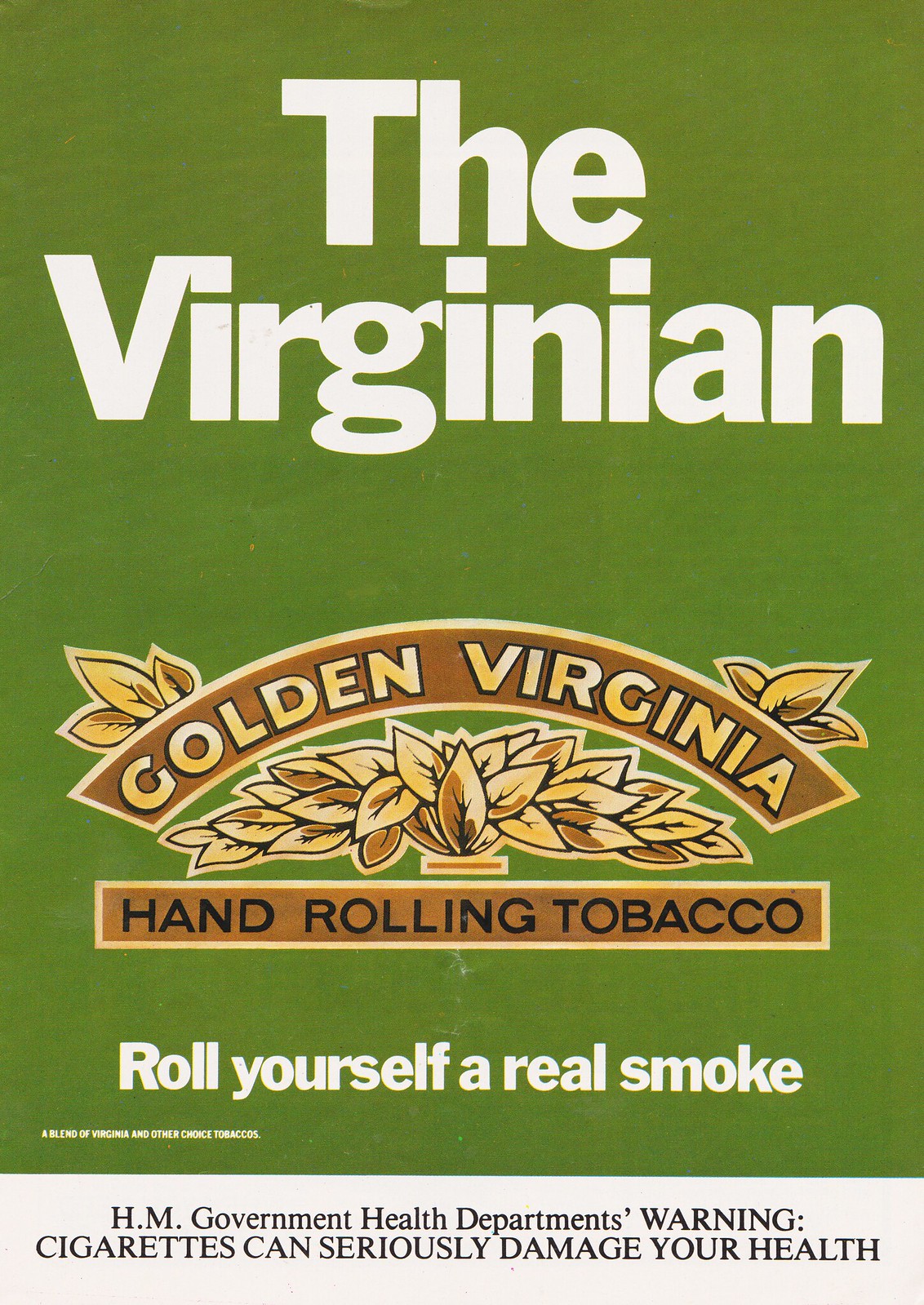The advertisement is a portrait-oriented vintage ad featuring a green background with multiple text elements in contrasting colors. At the top, bold white letters prominently display "The Virginian," with "Virginian" centered beneath "The." Below this is a brown banner outlined in gold, featuring bold yellow letters that say "Golden Virginia." Flanking this banner are illustrations of golden tobacco leaves. Directly under the "Golden Virginia" banner is another brown rectangle with a gold outline, and black text that reads, "Hand Rolling Tobacco." Centered below this in bold white letters is the phrase "Roll Yourself a Real Smoke." At the bottom of the ad, a white footer in black print states, "HM Government Health Department Warning: Cigarettes can seriously damage your health." The overall layout and the wording of the health warning suggest that this is an old advertisement for rolling tobacco. Additionally, there is small white text in the lower left-hand corner that reads, "A Blend of Virginian and Other Choice Tobaccos."